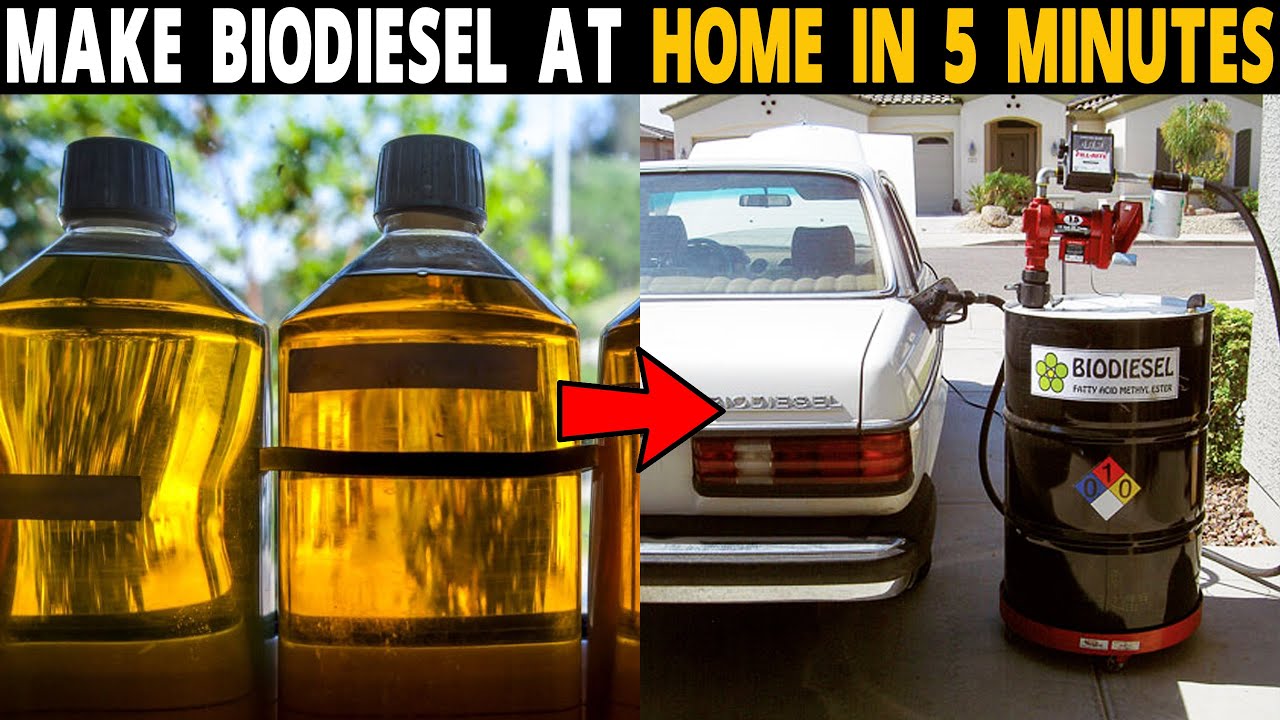The advertisement, captioned "Make Biodiesel at Home in Five Minutes," features white text and emphasizes the quick and easy process of producing biodiesel. Below this headline, the ad is split into two sections. On the left side, there are two jars filled with a yellowish-amber liquid, each sealed with black caps. A red arrow directs the viewer's attention to the right side, where an old white car is shown being fueled by a barrel labeled "biodiesel." The barrel, topped with a complex red contraption, efficiently dispenses biodiesel into the car. In the background, a Southwestern-style home adds context to the setting.